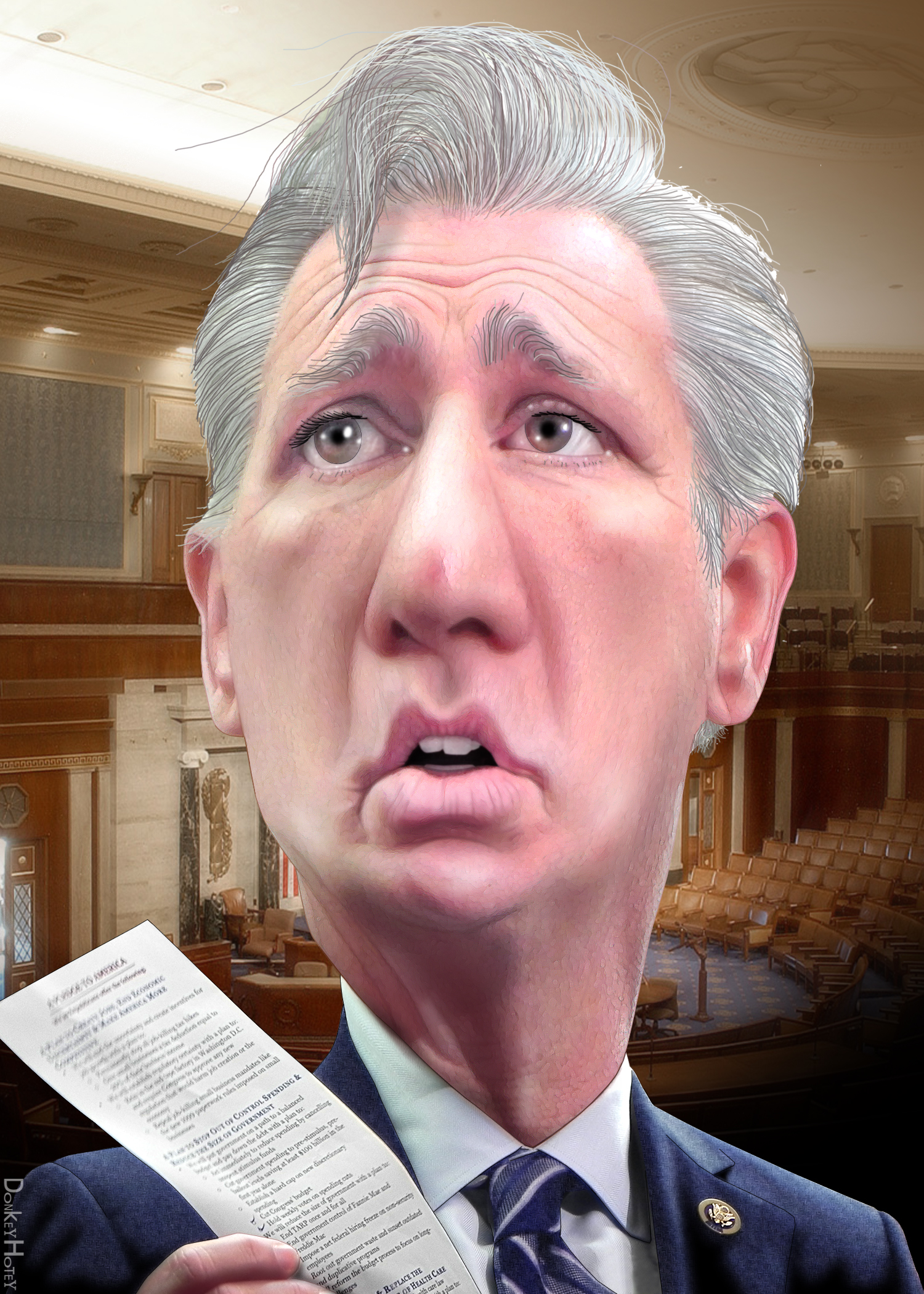This vertically aligned rectangular cartoon image is a satirical depiction of a Caucasian gentleman, seemingly a caricature of a figure in U.S. politics. The man's face is exaggerated and elongated, featuring short grayish-white hair, bushy eyebrows, and an unusually large nose. His expression is one of concern, indicated by his scrunched eyebrows, worried eyes, and slightly open mouth revealing his teeth. He is dressed in a navy blue suit jacket, a white collared shirt, and a striped blue and gray tie. The gentleman is holding a receipt-like piece of paper in his right hand, which appears in the lower left corner of the image. The background suggests a large political setting, possibly a congressional auditorium, with numerous seats and a floor designed for speaking engagements.